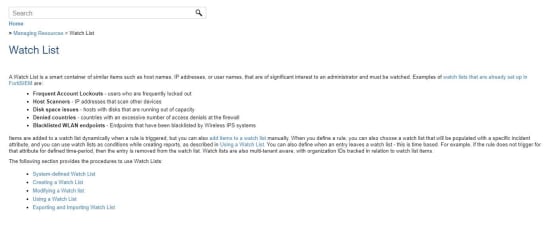This screenshot captures a portion of a web interface featuring a search bar situated within a magnifying glass icon. Directly beneath the search bar is the word "Home." The image also includes a blue clickable link labeled "Watch List." Below this link is a segment containing text, which is largely illegible due to its small font size. However, certain phrases can be discerned, including "IP address," "Frequent account lockout," "Home scanners," and "WLAN information," which are all in bold font.

Additionally, the image shows another paragraph before a section labeled "paid break." The paragraph seems to introduce the following segment which states, "The following section provides the procedures to use Watch List." This section is accompanied by five different blue hyperlinks that are presumably related to the procedures mentioned.